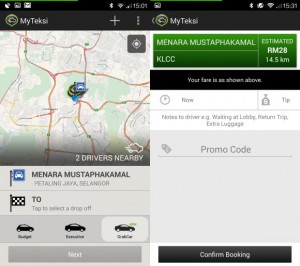The image depicts a smartphone screen displaying the "MyTeksi" application, a ride-hailing service similar to a cab booking app. The screen is divided into two sections showing different stages of the booking process. 

The top of the screen features a gray header with the app name "MyTeksi" written in white. The app's icon is a green circle enclosing a car. The status bar is visible, showing various system icons such as time (15:01 on the left screen and 15:31 on the right screen), Bluetooth, Wi-Fi, network signal, and screenshot.

On the left side of the screen:
- There's a map indicating the user's current location.
- Icons of MyTeksi cars are shown, signifying nearby available vehicles.
- A message states "2 drivers nearby."
- At the bottom, the text "Menara Mustapha Kamal" is displayed alongside an option to select a drop-off point.
- Users can choose the type of car they want (Budget, Premium, or GoCar).
- A button labeled "Next" is present to proceed with the booking.

On the right side of the screen:
- The text "Menara Mustapha Kamal" appears at the top, followed by an estimated fare of RM 28 for a distance of 15.5 kilometers.
- There's a space to add a promo code.
- At the bottom, a black button marked "Confirm Booking" is available to finalize the ride request.

The detailed interface captures the critical elements and functionalities of the MyTeksi app, providing a clear and intuitive experience for booking a ride.